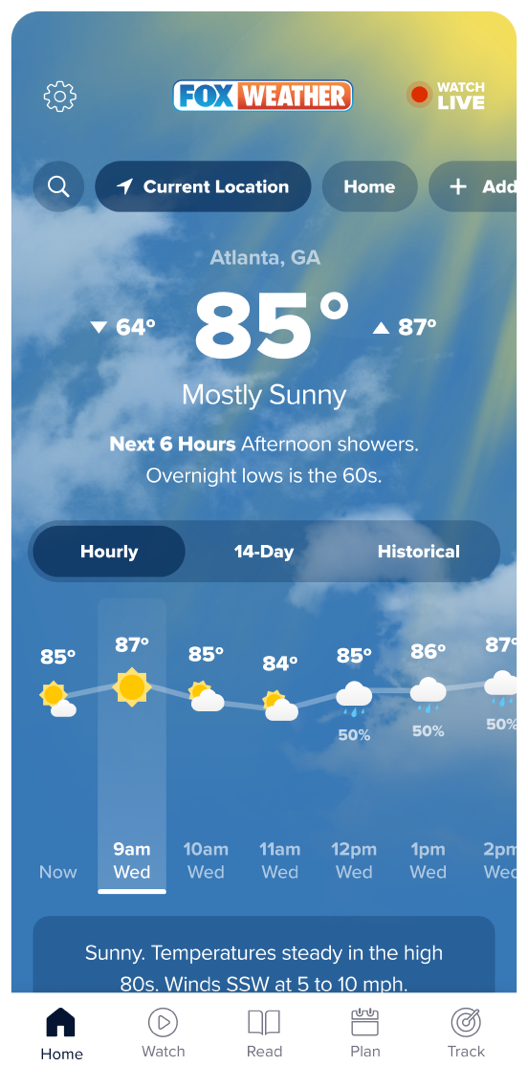This is a detailed screenshot likely taken from a smartphone, showcasing the Fox Weather app. The image features a rectangular format consistent with a smartphone display. Dominating the top-middle of the screen is an oblong box displaying the "Fox Weather" logo, with "Fox" in blue font and "Weather" in white font set against a red and white background.

The overall theme of the image is a serene blue sky adorned with scattered white clouds, and in the upper right corner, there is a yellow sun radiating sunbeams. The screen indicates the current weather for Atlanta, Georgia, revealing a temperature of 85 degrees Fahrenheit and conditions described as mostly sunny. The forecasted high and low temperatures for the day are displayed flanking the current temperature, with a high of 87 degrees on the left and a low of 64 degrees on the right.

Further down, the screen informs users about the weather for the next six hours, mentioning afternoon showers and overnight lows in the 60s. Below this information, there are tabs for "Hourly," "14 Day," and "Historical" forecasts, providing users with options to view more detailed weather data.

At the very bottom of the screen, there is a concise summary: "Sunny, temperature steady in the high 80s, winds south-southwest at 5 to 10 miles per hour."